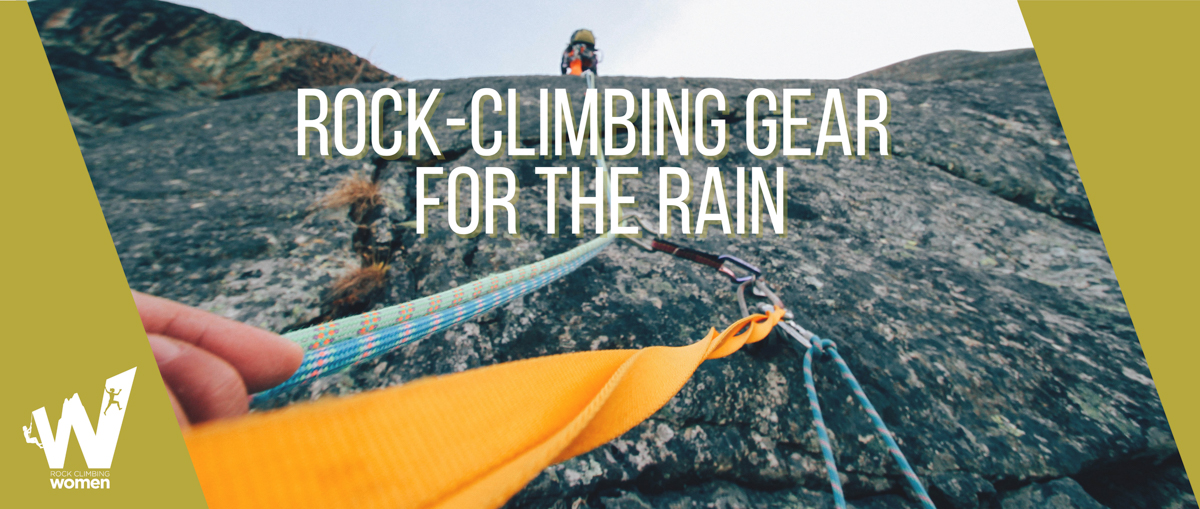In this advertisement for Women’s Rock Climbing Gear for the Rain, produced by a company starting with a W, the image prominently features an adventurous scene of rock climbing. The focal point is a woman scaling a massive, dark gray, and tan rock face, giving the viewer the impression of ascending the mountain themselves due to the sideways angle of the photograph. The determined climber, seen from behind and partially obscured by her climbing gear, is securely fastened with ropes and harnesses, her hand gripping the line tightly as she progresses upward. Above her, another climber is visible, nearing the mountain’s summit. The background showcases a dramatic landscape, with dark blue, wavy water reflecting white light, brown and green hues on a distant mountain, and a contrasting sky split between gray and white. Two dark yellow isosceles triangle-shaped barriers frame the scene, adding depth. In the lower left corner of the image, an emblem with a bold W and the word “Woman” reinforces the brand, and nearby text highlights “Rock Climbing Gear for the Rain” in large capital letters, marketing the specialized equipment featured.